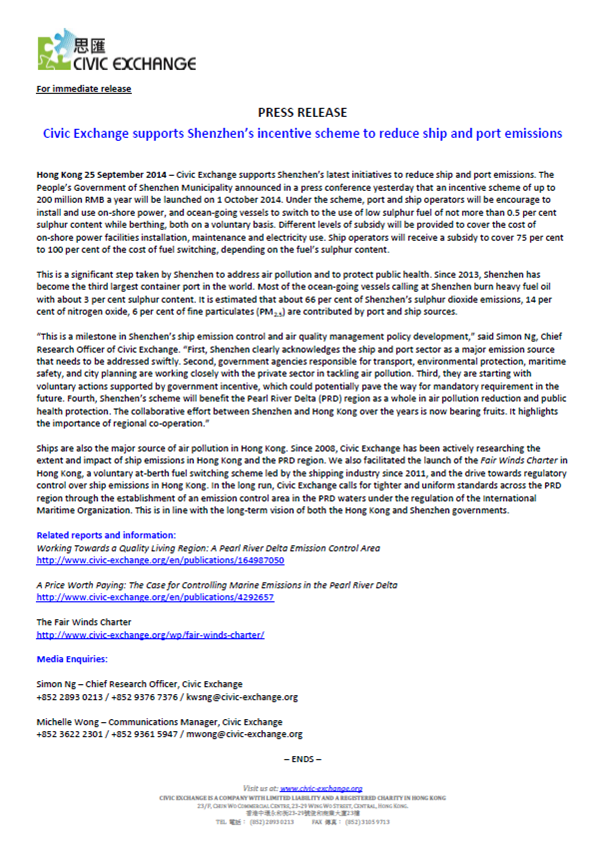**Detailed Caption for Screenshot from Civic Exchange’s Press Release:**

The screenshot displays a press release from Civic Exchange, featuring a green and blue icon that resembles puzzle pieces. The text includes non-English characters, possibly Korean, followed by "Civic Exchange" written in English. Dated 25 September 2014, the press release announces Civic Exchange's support for Shenzhen's incentive scheme aimed at reducing ship and port emissions, set to launch on 1 October 2014.

**Key Highlights:**
1. **Support Announcement:** Civic Exchange commends Shenzhen's initiative to incentivize the reduction of emissions from ships and ports.
2. **Incentive Details:** The People's Government of Shenzhen Municipality will introduce an incentive scheme with an annual budget of up to 200 million RMB. This scheme promotes the installation of onshore power facilities and the use of low-sulfur fuel, encouraging voluntary participation from port and ship operators.
3. **Subsidies Offered:** Subsidies covering 75% to 100% of the costs associated with fuel switching and onshore power facilities will be provided, depending on the fuel's sulfur content.
4. **Environmental Impact:** The initiative targets significant emission reductions. Currently, the ship and port sectors contribute immensely to Shenzhen's sulfur dioxide (66%), nitrogen dioxide (14%), and fine particulate matter emissions (6%).
5. **Milestone Recognition:** Simon Ng, Chief Research Officer of Civic Exchange, highlights this incentive scheme as a milestone in Shenzhen's policy development for air quality and emission control.
6. **Regional Benefits:** This scheme is expected to have positive impacts on air quality and public health in the Pearl River Delta (PRD) region, benefiting both Shenzhen and Hong Kong.
7. **Civic Exchange’s Role:** Since 2008, Civic Exchange has been researching ship emissions in the Hong Kong and PRD region. They've facilitated the Fairwinds Charter in Hong Kong, promoting voluntary fuel-switching and pushing for stringent regulatory control.

**Contact Information for Media Inquiries:**
- **Simon Ng:** Chief Research Officer, Civic Exchange. Phone: +852-289-30213 / +852-9376-7376. Email: kwsng@civic-exchange.org
- **Michelle Wong:** Communications Manager, Civic Exchange. Phone: +852-3622-2301 / +852-93615-947. Email: mwong@civic-exchange.org

The press release underscores Shenzhen's commitment to environmental protection and highlights the collaborative efforts between Shenzhen and Hong Kong, aiming for long-term improvements in regional air quality. 

**Additional Resources:**
- Links to key reports and information related to PRD emissions control and the Fairwinds Charter are provided below the main text. Some text at the bottom is not readable.